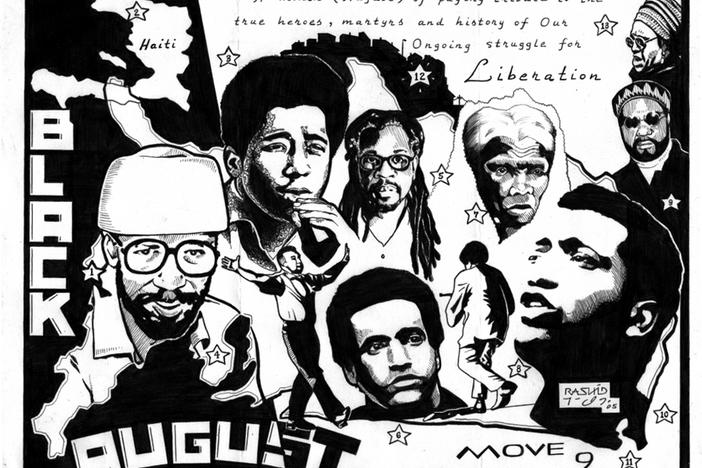This black and white mural prominently features the text "Black August" on the left side, written in white font, signifying its dedication to Black August, a month that commemorates Black resistance. At the bottom, it displays the words "Move 9." The mural is rich with historical context, depicting the ongoing struggle for liberation with the phrase "true heroes, martyrs, and history of our ongoing struggle for liberation" prominently visible at the top.

Central to the artwork is the country of Haiti, indicating its significant role in Black liberation. The mural showcases various iconic Black figures: a man with a white hat and glasses adorned with a star pin on his chest, a man with an afro, and another with long dreads. Another notable figure appears to be speaking with "Rashid" signed near his neck area. In total, there are about 10 individuals, each representing different facets of the Black liberation movement.

The figures include a man wearing a traditional Jamaican-style hat, another in sunglasses with a cultural hat, and a figure with rough ridges on the eyebrows resembling a Neanderthal, symbolically representing different periods or aspects of struggle and activism. These diverse representations collectively emphasize the mural’s theme of resistance, resilience, and the historical importance of Black August.